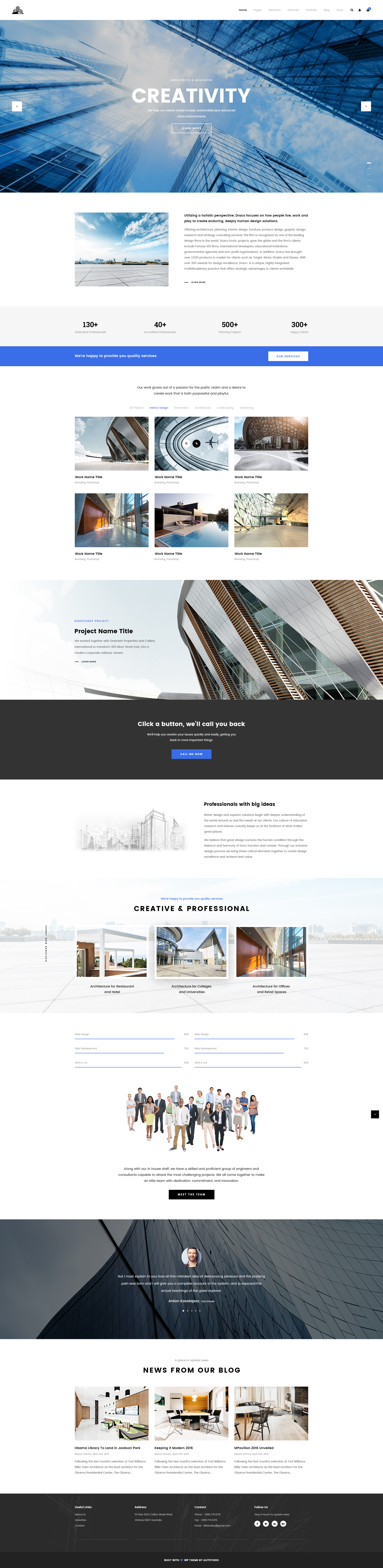A detailed screenshot of a website is depicted. At the top, there is a small graphic resembling a building. To the right of this graphic, a navigation bar lists links labeled Home, Pages, Elements, Features, Portfolio, Blog, and Shop. An icon of a magnifying glass represents a search function, and a person icon appears beside an email link. The text for "Home" is emphasized in a darker black font, indicating the current page.

Beneath the header, a larger graphic showcases an upward view of a building stretching towards the sky, accompanied by the text "Creativity and Wayprint" and "Architects and Associates." A small tab labeled "Learn More" is also visible.

Scrolling further down, the background turns white, featuring an image of a distant sky and buildings. A headline reads "Utilizing a Holistic Perspective," followed by a description of Draco's approach to design, focusing on lifestyle elements to create lasting and human-centric solutions. Another "Learn More" tab is presented beside this section. Notable statistics are highlighted: "130+ Dedicated Professionals," "40+ Accredited Professionals," "500+ Planning Projects," and "300+ Happy Clients."

The next section showcases the firm's passion for the public realm and the creation of work that balances purposefulness and playfulness, set against another clean, white background. There are six images arranged in two rows of three. Following this, project details are introduced under the heading "Project Name Title."

A prominent black banner states "Click a Button, We'll Call You Back," with a blue tab for "Call Me Now." The following section highlights "Professionals with Big Ideas" with a drawing of a cityscape.

The content continues with a declaration, "We're Happy to Provide Quality Services, Creative and Professional," next to additional images. The page concludes with an image of a cohesive group of people, suggesting collaboration and team spirit.